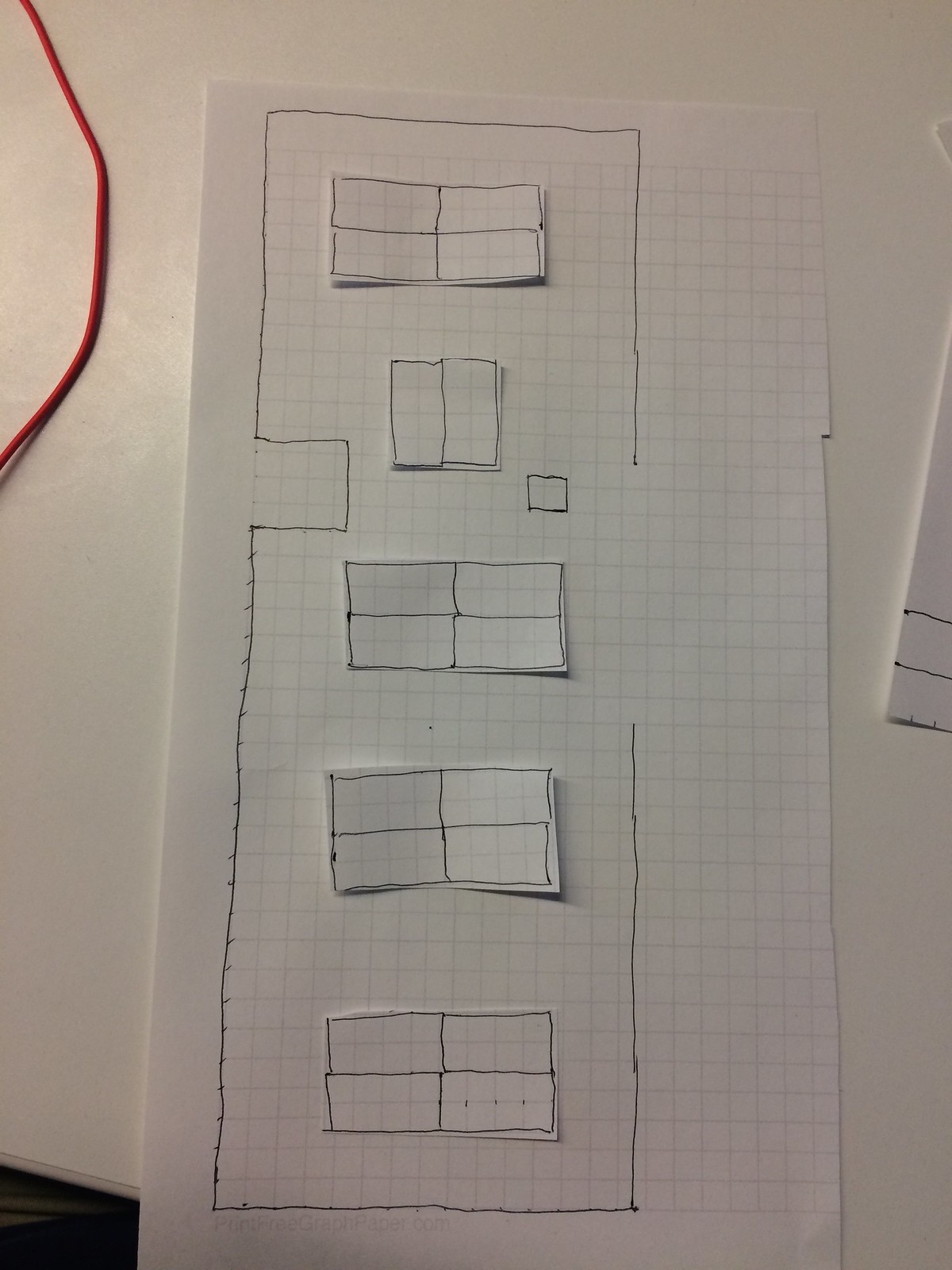The image showcases an intricate engineering design on graph paper, placed prominently at the center. Surrounding the design are cut-out shapes layered on top of the graph paper, contributing to the detailed visual representation. A red wire is noticeable in the top left corner of the image, adding a splash of color to the scene.

The focal point of the design resembles a high-rise building sketched in pen. The top section features a drawn square shape. In the middle of this square, there is a horizontally-oriented rectangular window. Directly beneath this is another square bisected by a horizontal line. To the right of this configuration lies a tiny square, while to the left, a distinctive notch interrupts the outline of the building.

Further down the design, there are three elongated, horizontally-aligned rectangle windows, each consisting of four panes. An incomplete section on the right side of the building’s middle part, where pen lines fail to meet, suggests an opening or unfinished area. The detailed line work and precise geometric shapes underscore the meticulous nature of the engineering design.